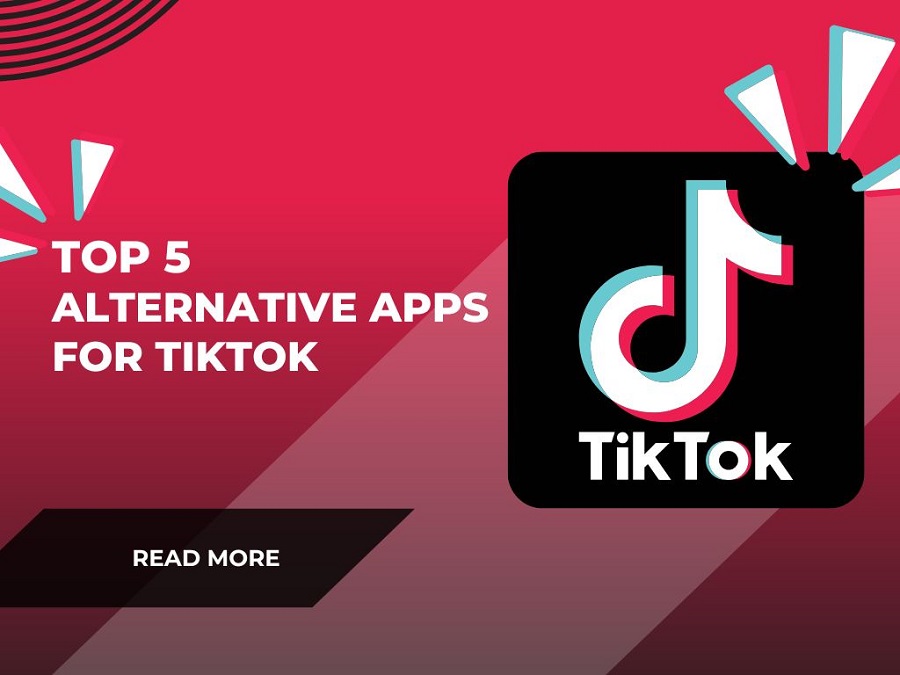This image serves as an advertisement for alternative apps to TikTok. Dominated by a striking red, pink, and maroon diagonal background, the design in the upper left-hand corner features black curved lines and a prominent black square containing the word "TikTok" in white letters. Next to the text is the recognizable TikTok musical note in the brand’s signature colors of green, white, and pink, with long, triangle-shaped extensions in matching colors emanating from the note.

On the left side, large white text reads, "Top Five Alternative Apps for TikTok," accompanied by additional triangles extending from the text. Below this, a black box with diagonal sides contains the phrase "READ MORE" in bold, all-capital white letters. The simplicity of the design ensures that the iconic TikTok branding and the message about alternative apps stand out clearly. This image aims to inform viewers about available alternatives in case TikTok becomes unavailable, rather than promoting TikTok itself.